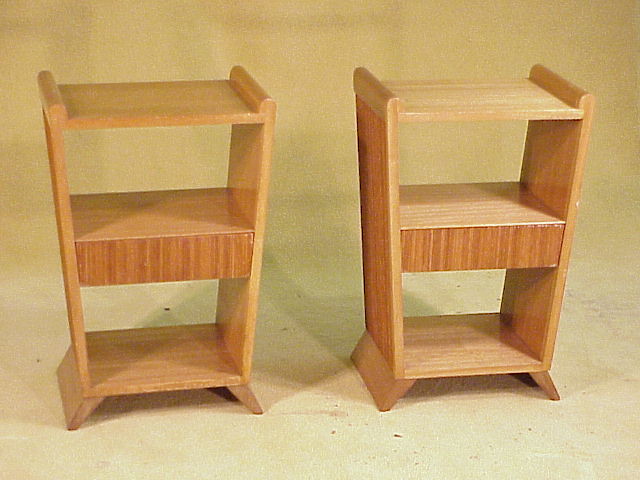The photograph depicts two identical wooden bookshelves, placed side by side with a small gap between them. Crafted from polished timber, each bookshelf has a shiny finish with a distinctive dark brown color in the middle segment. Both shelves, the same size and color, are designed with two open storage compartments and supported by two splayed legs at the bottom. There are no closing lids for these shelves, allowing open access from the front to the back for convenient storage. The sides of each bookshelf taper slightly narrower at the bottom and widen towards the top, with the side boards protruding slightly on the upper shelf. The mustard-colored background and matching floor highlight the bookshelves' medium brown hue, making these pieces suitable as bedside tables or kitchen storage solutions.